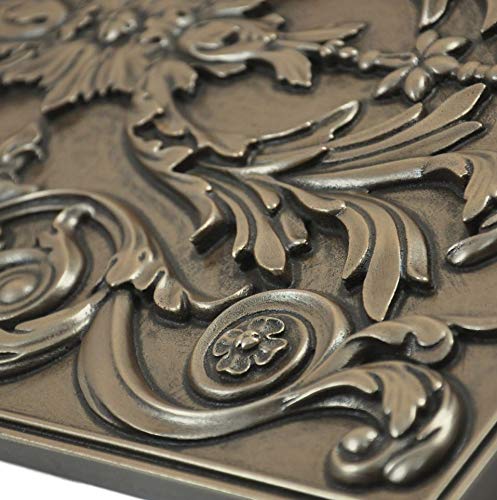This is a highly detailed close-up photograph of a piece of decorative bas-relief work in bronze, possibly part of a frame or a plaque. The image focuses on intricate engravings of botanical forms with flowing accents, akin to French Feudalese designs. Dominating the foreground is a prominent swirling motif with a flower at its center, surrounded by various raised leaf patterns and rosettes. The bronze surface has a subtle, polished patina, highlighted by darker accents in the recessed areas, enhancing the dimensionality and richness of the design. The background features more of these ornamental shapes, although they are slightly blurred to emphasize the central floral element. There is no text within the image, allowing the elaborate, almost heraldic decorations to stand out.